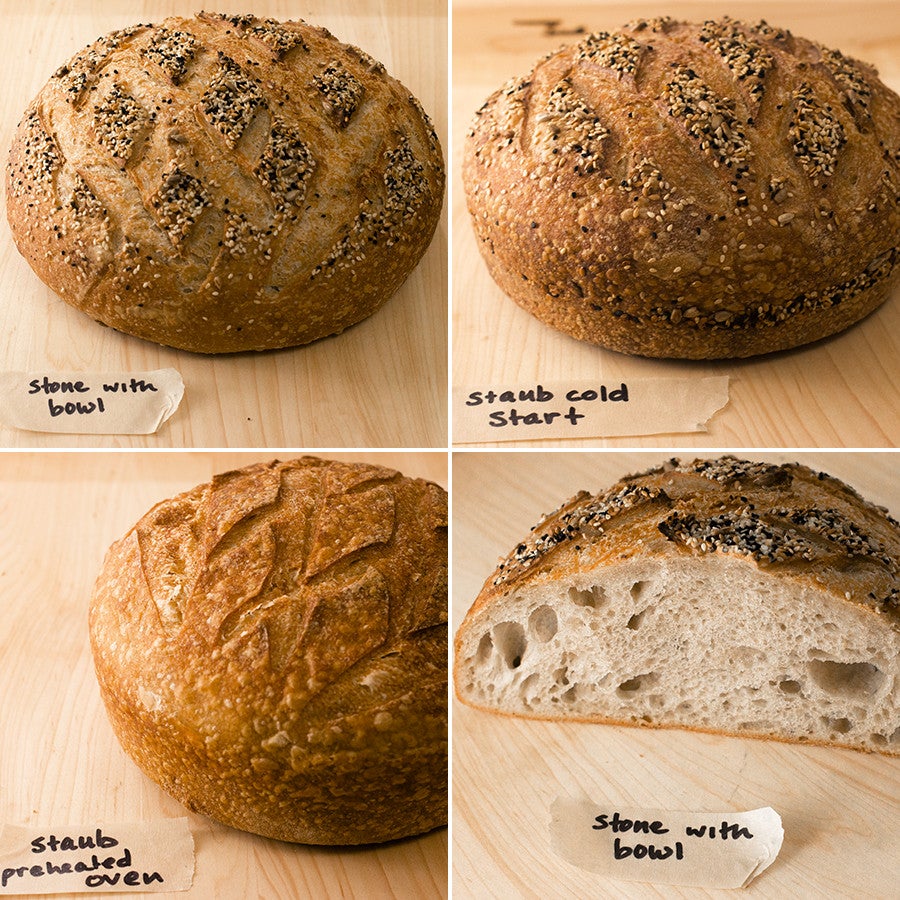The image is a panel featuring four different photographs of round loaves of bread or muffins, each on a light-colored wooden surface. The top left photograph shows a seeded muffin with a label that reads "stone with bowl." The top right photograph features a similar seeded muffin, labeled "Staub, cold start." In the bottom left quadrant, another muffin without seeds is labeled "Staub, preheated oven." The bottom right photograph depicts a cut muffin, revealing its interior with a label that also says "stone with bowl." Each label in the image indicates a different baking method, illustrating the outcomes of baking bread using varying techniques.